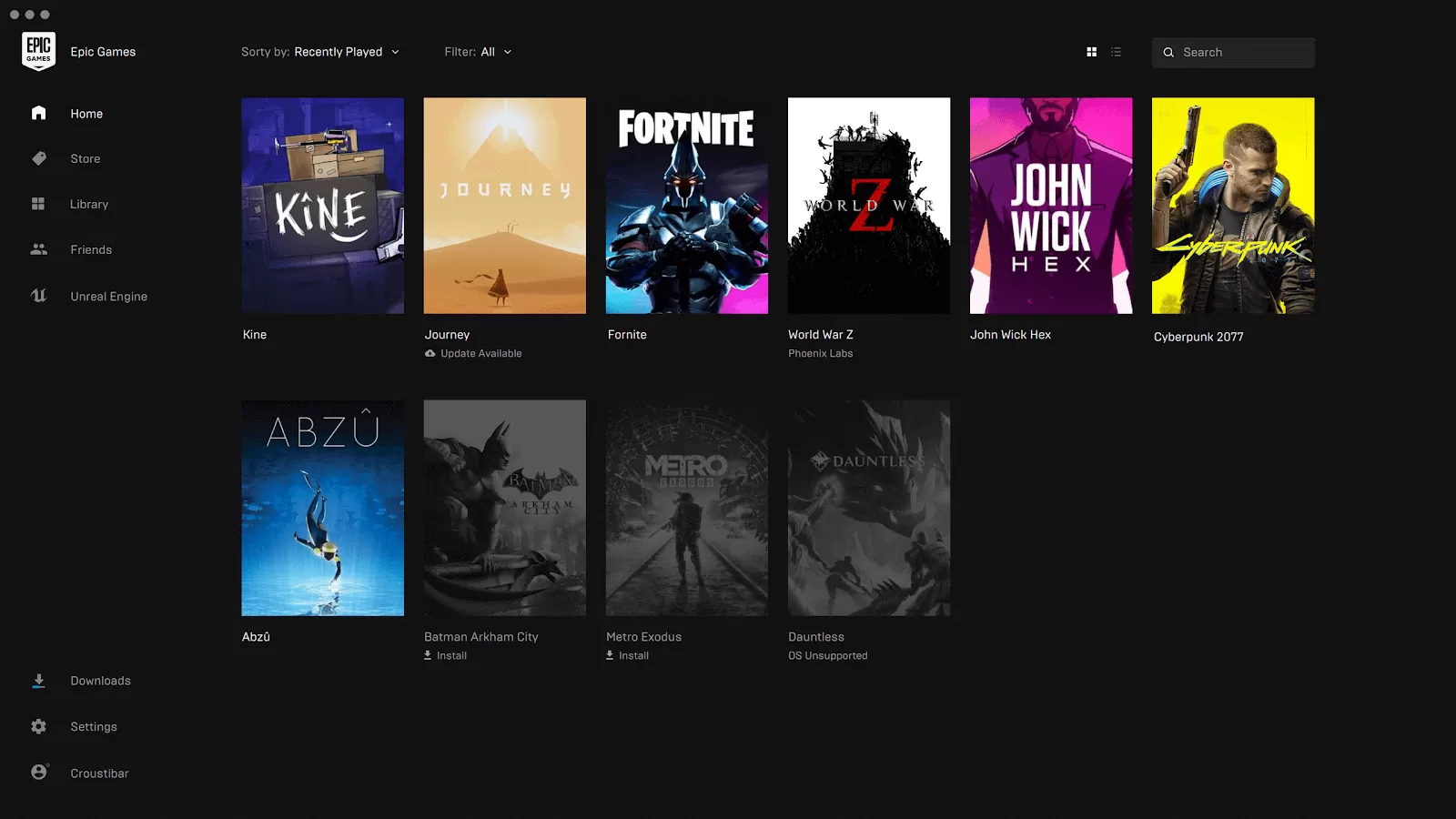The image depicts a sleek, black, horizontal web page belonging to C.O.C. Games. The top heading reads "C.O.C. Games," accompanied by a small logo that includes the word "Epic," indicating the platform might be associated with Epic Games. The content is organized under the heading "Sorted by Recently Played," confirming that the items displayed are games. 

This page features thumbnail images of various games arranged in a grid format. The highlighted thumbnails, marked with numbers 1, 2, 3, 6, and 7, signify the games that the subscriber has recently played. The games include titles such as "Kine," "Journey," "Fortnite," "World War Z," "John Wick Hex," "Cyberpunk," and "ABZU." The thumbnail for "ABZU" illustrates an individual diving, likely portraying an underwater adventure, although it could also suggest aerial diving.

Below the highlighted games are three more categories that are not illuminated, suggesting these are additional games that the subscriber has yet to explore or select.